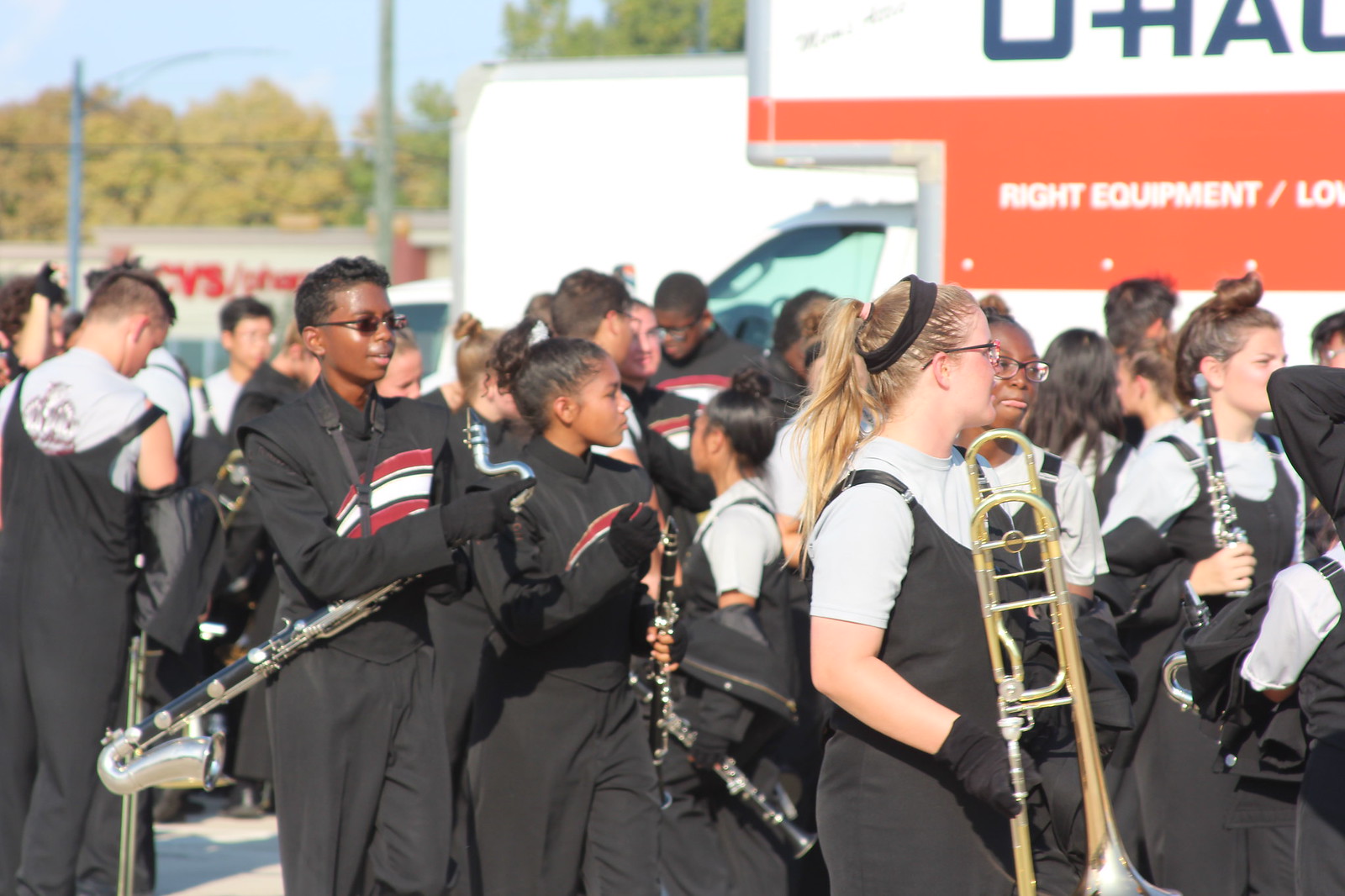The photograph captures a group of high school teenagers, likely aged between 14 and 17, gathered in a parking lot, presumably for a band practice or prior to a performance. The band members are dressed in various stages of their uniforms; some wear white or gray t-shirts with black coveralls, while others don more formal tops featuring a distinctive red and white curvy stripe pattern. Many also sport black gloves and a few have accessories like headbands. The diverse group, comprising both males and females of varying ethnicities, is seen holding a variety of musical instruments including trombones, clarinets, and a possible saxophone. Notably, a girl with a ponytail and glasses stands at the forefront holding a trombone. In the background, a U-Haul truck marked with "Wright Equipment" and a CVS pharmacy are visible, along with some light poles and trees, situating the scene in what appears to be a school or event parking lot.